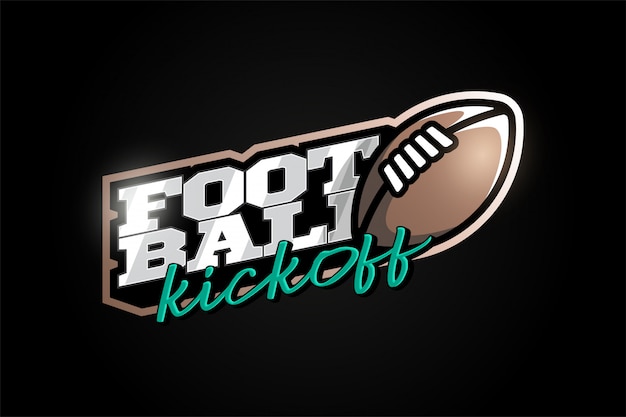This image depicts an artistic advertisement featuring the text "Football Kickoff" and a graphical representation of a football. Set against a solid black background, the composition is centered, with "Football" written in big, bold white letters. Directly beneath it, the word "Kickoff" is displayed in a greenish, cursive font. To the right of this text, there is a detailed drawing of a football, shaded in brown with prominent white stripes on its top portion. The football itself is angled upwards, pointing towards the top right corner. The entire scene is outlined slightly in brown, giving it an added dimension. The minimalistic design and color palette, which includes blacks, whites, brown, gray, and a dark mint green, draw attention to the focal point, making it an effective advertisement for a football event.